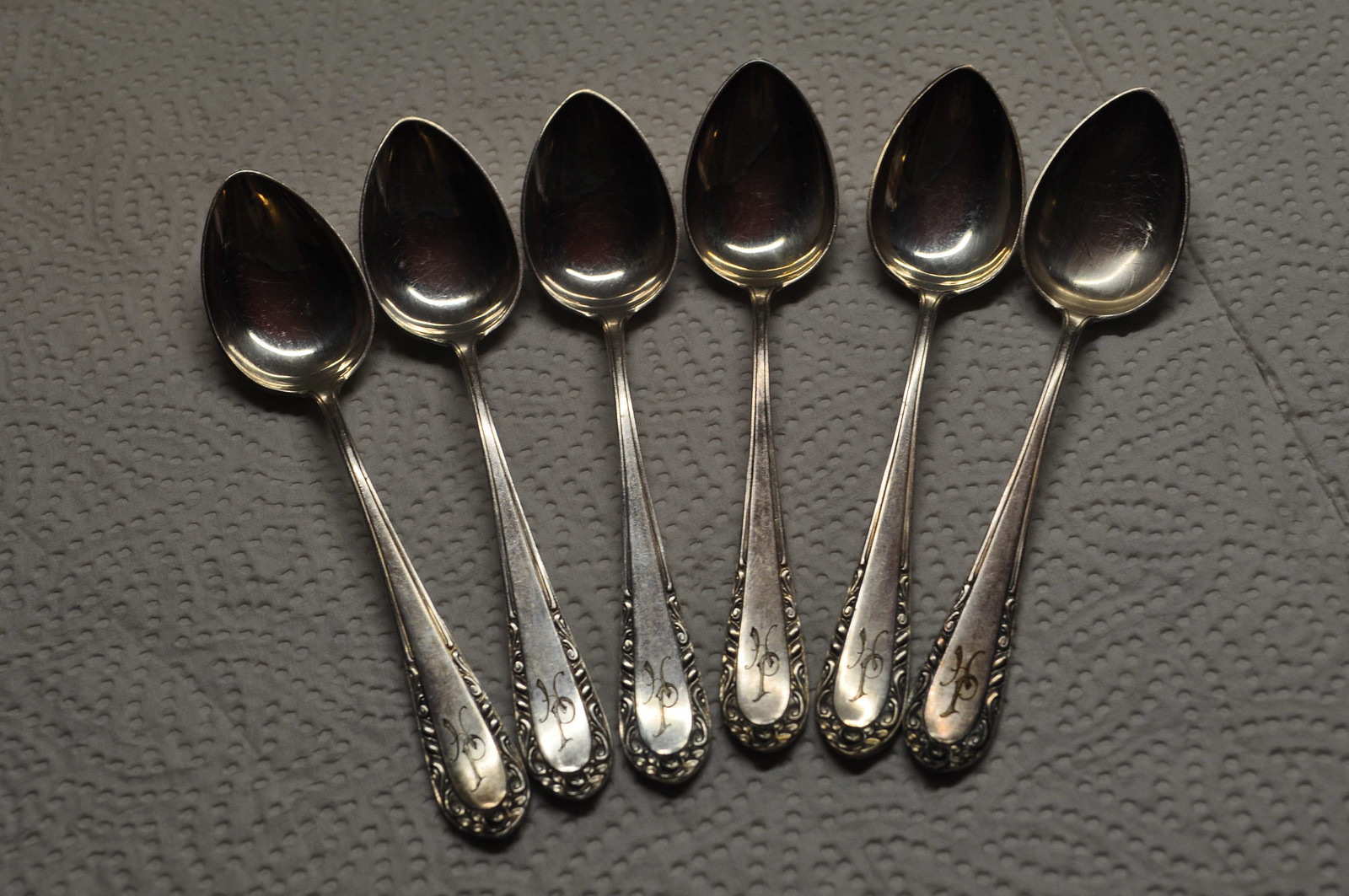This is a photograph taken from an angled, overhead view of six polished silver spoons laid out side by side on a white paper towel with an embossed pattern. The spoons are of uniform size and are positioned with their handles pointing downward, creating a slight arch-like arrangement. Each spoon's handle features a light floral engraving around the tip, and at the very end, there is an engraving of the initials "HP." Despite the soft, dark lighting of the image, reflections of light are visible in the bowls of the spoons, highlighting their polished surfaces. The spoons show minor signs of wear, adding character to their ornate design.